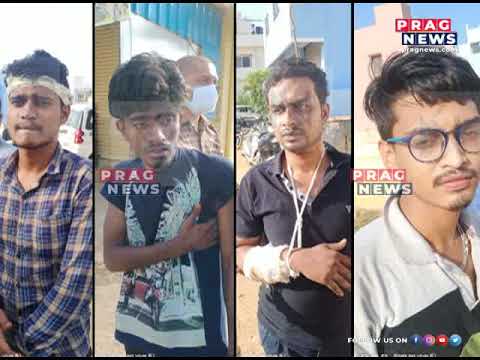The image resembles a poster with a predominant red background and a central white area. The colors are haphazardly blended, creating a distressed visual effect. In the top left corner, a troubling scene depicts a woman with black hair, wearing a white t-shirt, being forcibly held down by an unseen assailant. On the opposite side, the upper right, there is an illustration of a distraught woman with medium to long black hair, donning a torn red dress, and covering her face with both hands, indicating distress. Above this illustration, the text "PRAC News" is displayed. Foreign text, written in non-Roman characters, occupies the center of the image, and at the bottom, there's a prompt to "follow us on," accompanied by the icons for various social media platforms, including Facebook, Instagram, YouTube, and Twitter/X. The overall style suggests it's an advertisement or public service announcement.